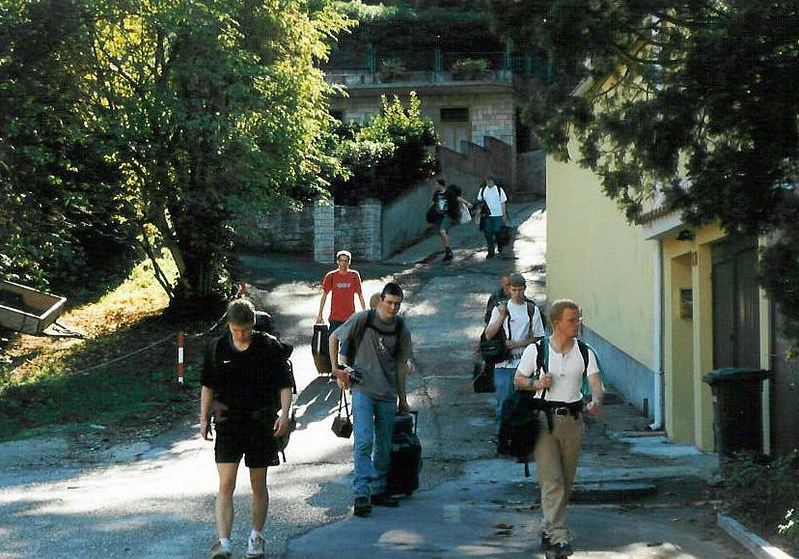A horizontally aligned rectangular photograph captures a group of young men, possibly on a study abroad program in the 90s, walking towards the camera, up an old, cracked cement street. They all carry various pieces of luggage: the man on the left wears black shorts and a black short-sleeve shirt with a large backpack; the one in the center sports a baggy gray t-shirt and jeans, holding a handbag, a backpack, and a piece of luggage with a handle; and the man on the right dons khaki pants and a tight white shirt, carrying a black bag over his shoulder and a backpack. The group appears to be heading up a hill, possibly in Europe. On the right side of the image stands a building with a gray cement base and a yellow (or faded beige) upper section, featuring two brown doors and a gutter running down its side. A residential garbage can is placed near the doorway. To the left, a large tree extends its green leaves over the walkway, and a fenced-off wooded area houses a wheelbarrow. Additional people, roughly five to ten in total, trail behind the main trio, all engaged in the same journey. At the center background, an older gray stone building is visible, enhancing the photograph's timeless feel.